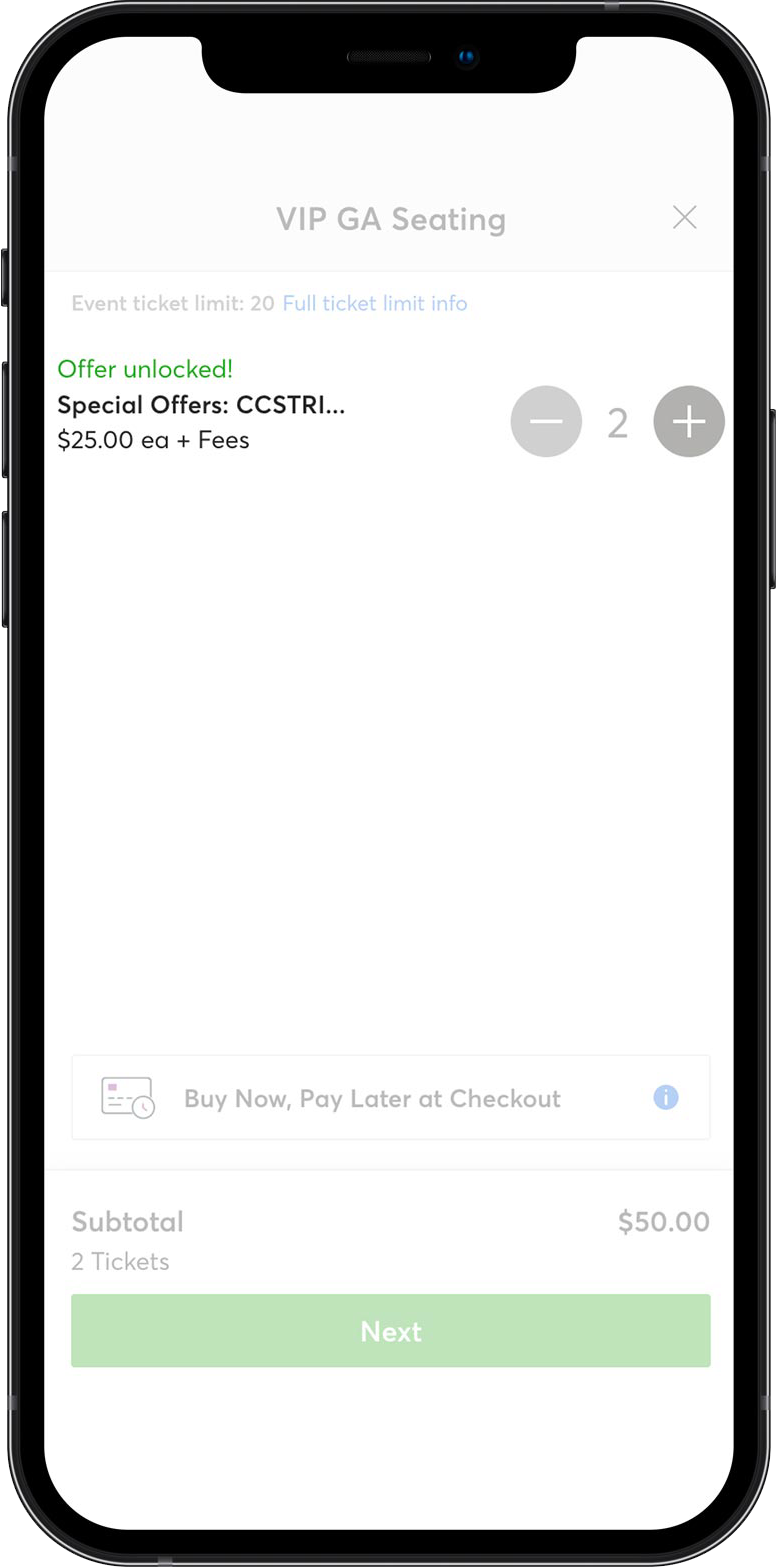The image depicts a website interface for purchasing event tickets. At the top of the page, there is a header displaying "VIP GA Seating." Below this, in small fine print, it states "Event Ticket Limit 20," "Full Ticket Limo," and "Limit Info." The background of the interface is predominantly white, but there are several green elements. A green notification reads "Offer Unlocked," followed by "Special Offers CC STRI" and a price of "$25 each." The user has selected to purchase 2 tickets, which is reflected in a subtotal of $50. Additionally, there is a message indicating the option to "Buy Now Pay Later at Checkout." Toward the bottom of the screen is a sage green box labeled "Next," guiding the user to proceed with the transaction.